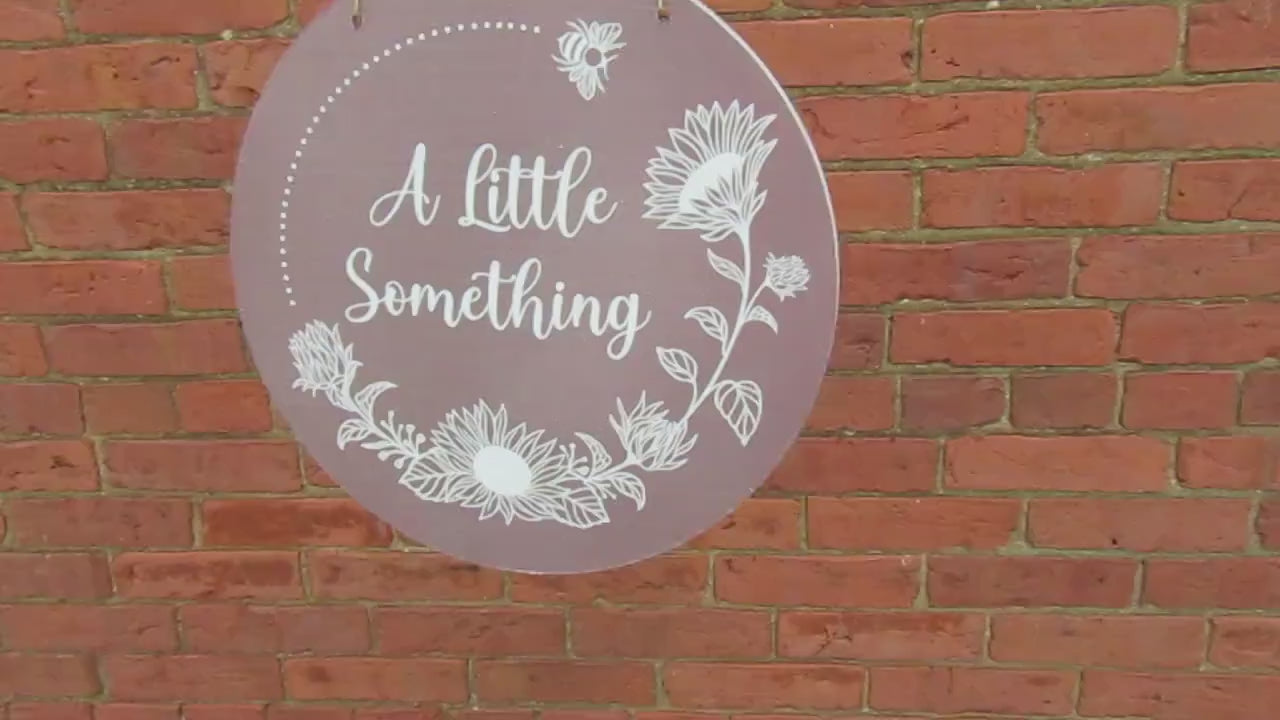The photograph depicts a red brick wall with a circular sign hanging from hooks. The sign has a lavender hue and features various floral outlines, including sunflowers and other flowers, etched in white along the bottom. A cartoon-like bumblebee is also etched in white. In the center of the sign, in cursive white lettering, it reads "A Little Something," likely indicating the name of a shop. The simplicity of the sign against the plain brick wall draws attention to its whimsical and inviting design.